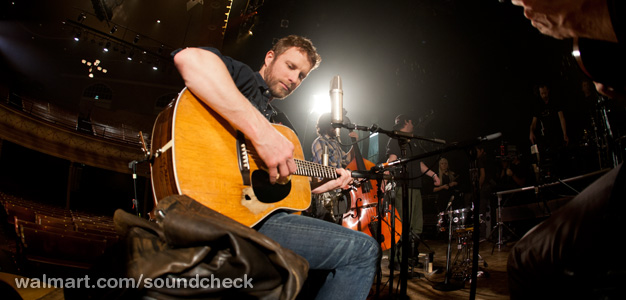A live performance image from Walmart.com/Soundcheck showcases a guitarist on stage, potentially the lead act, identified by the microphone stand positioned in front of him. He is dressed in blue jeans and a black polo shirt, has short brown hair, a beard, and is playing an acoustic guitar while seated. The stage is populated with various instruments, including drums and what appears to be an acoustic bass being played by another musician in gray pants and a black shirt. The background is predominantly dark, with some colored lighting creating a dramatic effect. The setting appears to be inside a performance hall or theater, possibly with an audience, although no crowd is distinctly visible. The guitarist is captured in a moment of concentration, looking down as he strums, with sideburns framing his face, all under the subtle watermark indicating the promotional nature of the image.